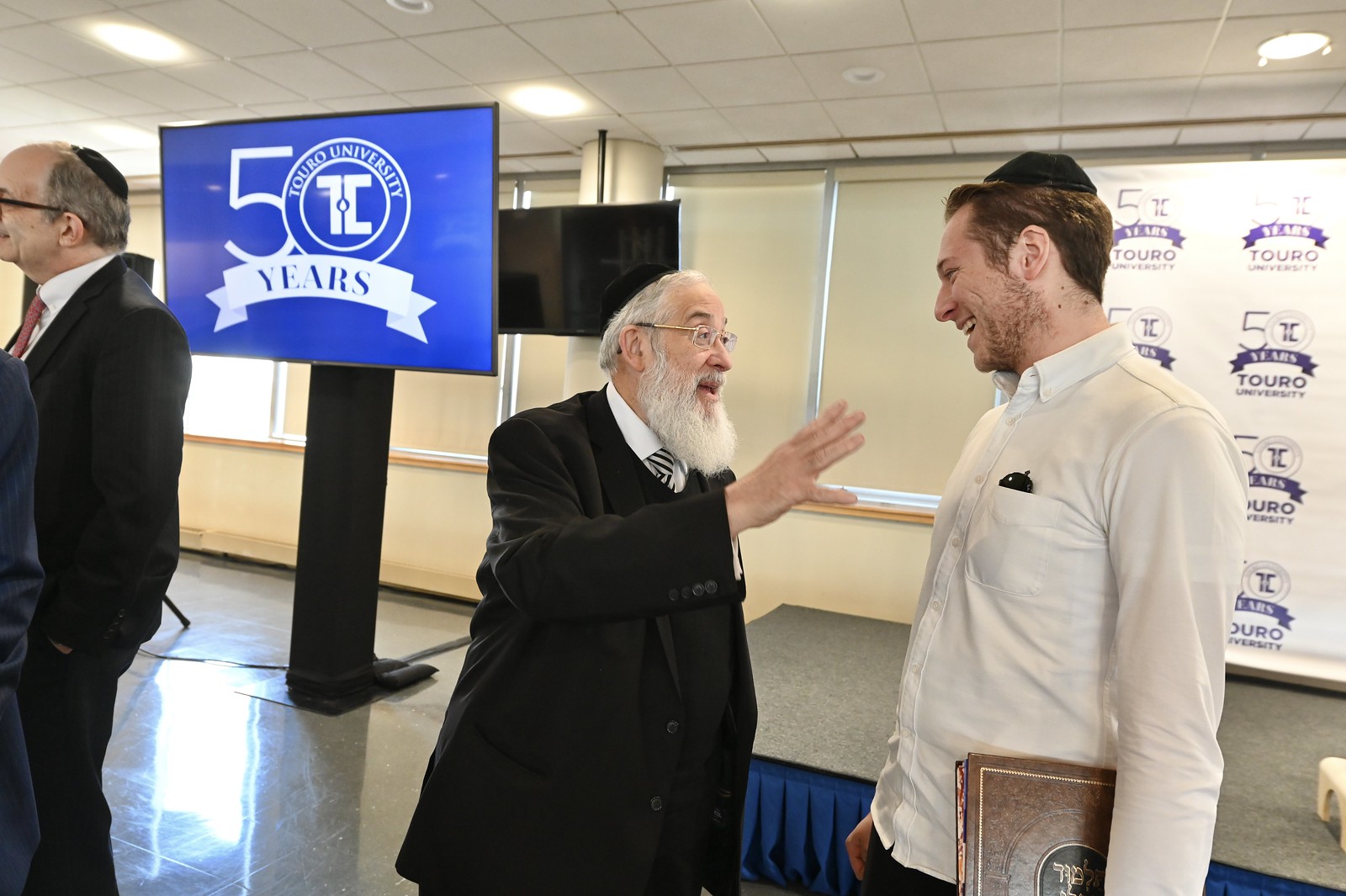The photograph captures an indoor ceremony at Toro University, commemorating its 50th anniversary. At the center, an older man with a large white beard, wearing glasses, and dressed in a black suit with a white shirt, engages animatedly with a younger man. This younger man has dark brown hair, a slightly unshaven face with a bit of a beard, and is dressed in a white long-sleeved collared shirt with a black cap (yarmulke) perched on his head. He holds a brown book featuring a black circle in the middle. Both men are smiling warmly at each other. The older man is gesturing expressively with his hand, extending three fingers towards the younger man's face and his pinky towards his chest. 

Behind them, a large TV set on a black stand displays a white backdrop with the text “50 years Toro University.” Another black screen hangs on the wall behind it. To the left, partly out of the frame, stands another man in a black suit, with a receding hairline, gray hair, and a black cap. The room features a tiled ceiling, glossy gray floor, and white walls that emphasize the predominantly white, black, and blue color scheme of the event. This detailed setup, complete with men wearing traditional yarmulkes, underscores the Jewish cultural context of the celebration.